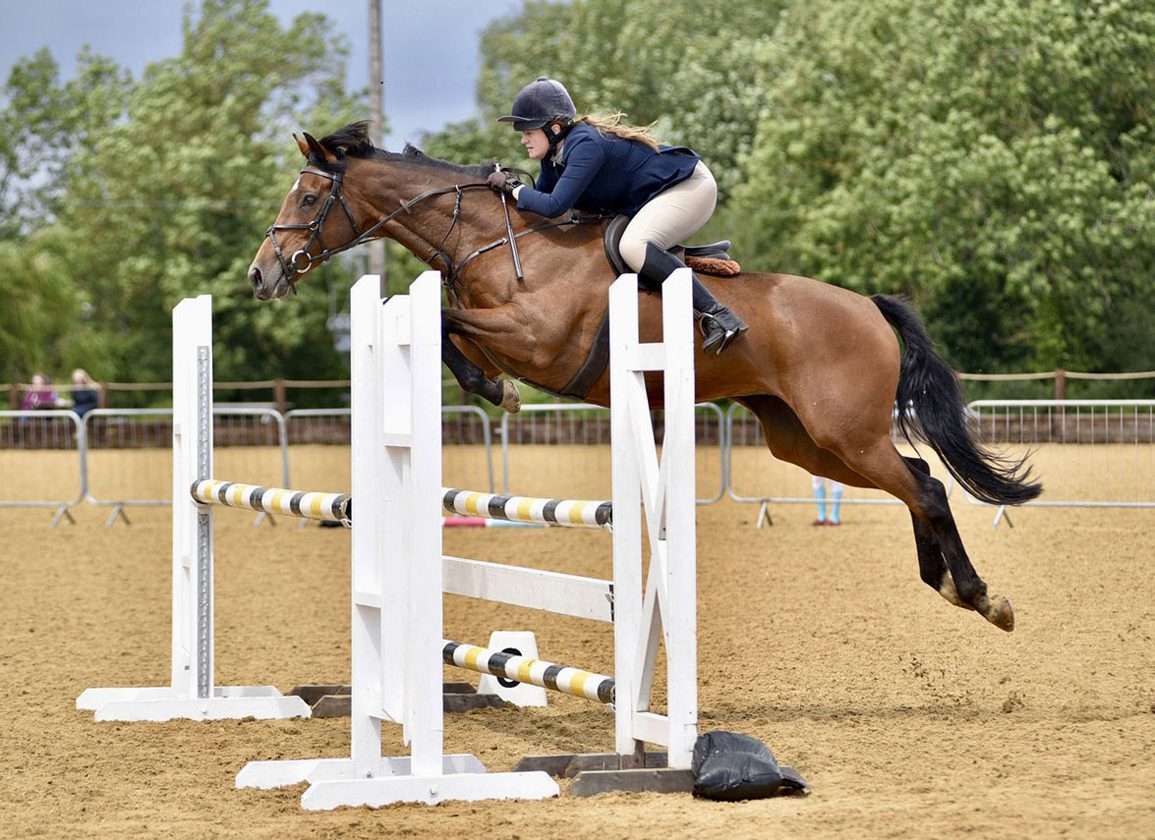In this captivating photograph, a female equestrian, a young woman with long blonde hair tucked under a blue riding helmet, is captured in a dynamic mid-air jump on her beautiful brown horse with a black tail. Both the rider and the horse are shown in perfect harmony, as they soar over two closely spaced bars that are striped in white, yellow, and black, supported by white stands. The rider is dressed in the quintessential equestrian attire: a blue blazer, tight white pants, knee-high black riding boots, and black gloves, embodying grace and precision. The horse is fully airborne, showcasing the power and elegance of both the animal and its rider.

The background sets the scene in what appears to be an equestrian park, with light brown dirt or sand covering the ground and white fencing outlining the area. Multiple trees, blurred but distinctly green, frame the background, along with a glimpse of a soft, cloudy sky in the upper left corner. Adding a touch of human element to the frame, two observers are visible in the distance, one dressed in purple and the other in blue, likely watching intently as the horse and rider execute their impressive jump. The composition and lighting suggest that this moment is either part of a training session or a competitive event, beautifully frozen in time by the photographer.